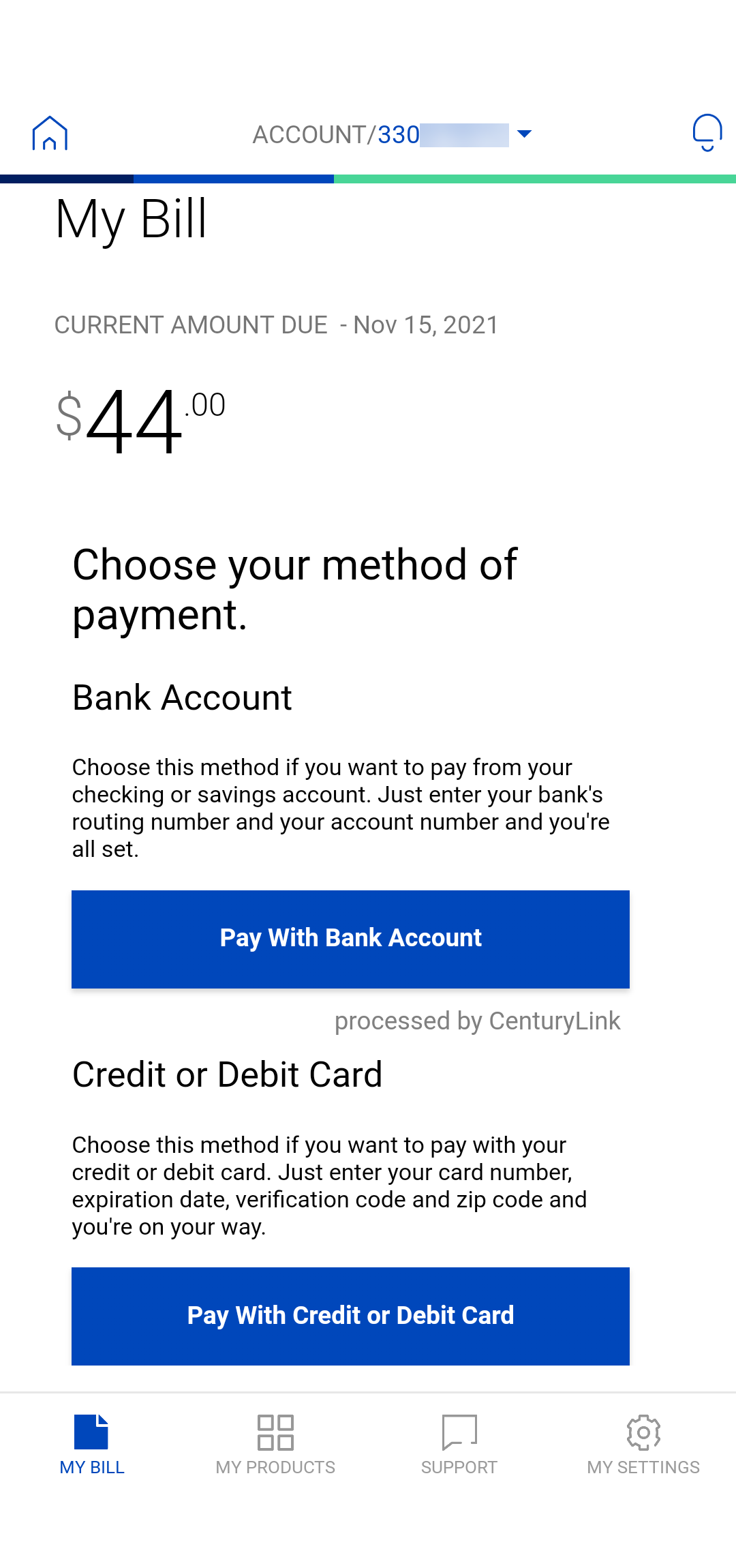The image features a white background with a variety of elements including text, icons, and buttons, arranged in a well-organized manner to display billing information and payment options. 

At the top center, there is a small blue house icon adjacent to the text "My Bill" in light blue. Next to it, there's a numerical count "1/330" inside a light blue box, followed by a downward arrow, likely indicating navigation or pagination options.

In the upper right corner, there's a semi-circle icon with a horizontal line beneath it and a small circle below that, possibly representing a user interface element.

Below these icons, a line transitions from black and blue to green, likely indicating progress or status.

The main section of the image contains text on a white background, structured as follows:

- In bold black print: "My Bill"
- Below it, in light blue print: "Current amount due: November 15, 2021"
- In black print: "$44.00"

Under the billing information, the text guides users on payment methods:

1. **Bank Account Payment Option:**
   - Text: "Choose your method of payment."
   - Sub-text: "Bank Account - Choose this method if you want to pay from your checking or savings account. Just enter your bank's routing number and your account number, and you're all set."
   - Large blue button with white text: "Pay with Bank Account"
   - Light blue text below button: "Processed by CenturyLink"

2. **Credit or Debit Card Payment Option:**
   - Text: "Credit or Debit Card - Choose this method if you want to pay with your credit or debit card. Just enter your card number, expiration date, verification code, and zip code, and you're on the way."
   - Large blue button with white text: "Pay with Credit or Debit Card"

At the very bottom, a navigation bar is highlighted in blue with options: "My Bill," "My Products," "Support," and "My Settings."

This detailed layout ensures users can easily understand their billing details and available payment options, making the process clear and user-friendly.